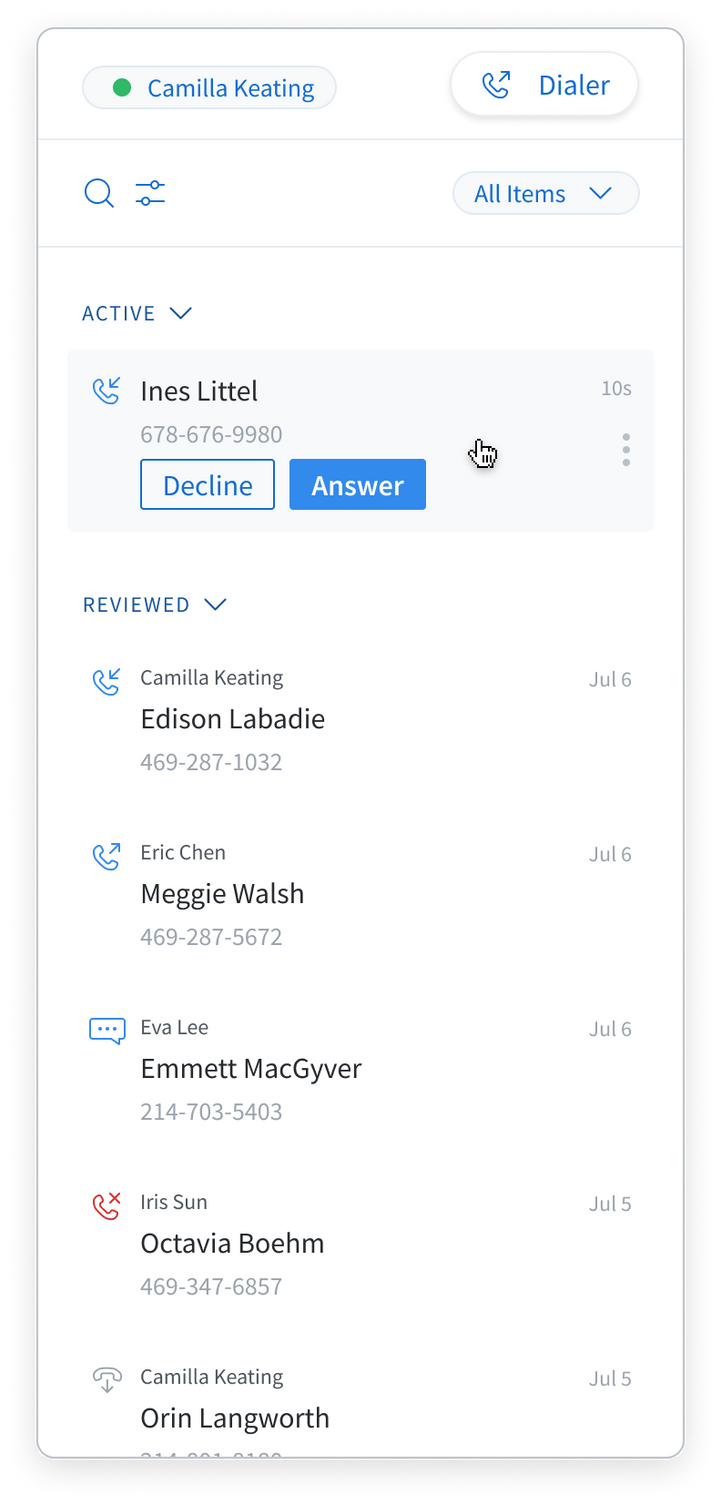The screenshot captures a call log within a communication app, likely resembling Skype, indicated by the interface elements. In the top left-hand corner, the user Camilla Keating is shown as online, marked by a small green dot next to her name. Adjacent to this, a phone icon with an arrow pointing outward labeled "Dialer" is visible, suggesting that clicking this icon will bring up a keypad for dialing calls.

Directly below this icon, there's a magnifying glass for search functionality, a button presumably for toggling or filtering options, followed by a drop-down menu labeled "All items."

In the main section of the screenshot, an active call is displayed, showing that Camilla is currently being called by someone. Two options are presented: a blue "Answer" button and a white "Decline" button. 

Below the active call section, there's a reviewed calls list. This list includes:
- Camilla Keating
- Edison Love, with the phone number 469-287-1032
- Eric Chin
- Emma
- Ava Lee
- Iris Son
- Camilla Keating again.

This detailed layout provides a clear depiction of the user interface and functionality within the app.